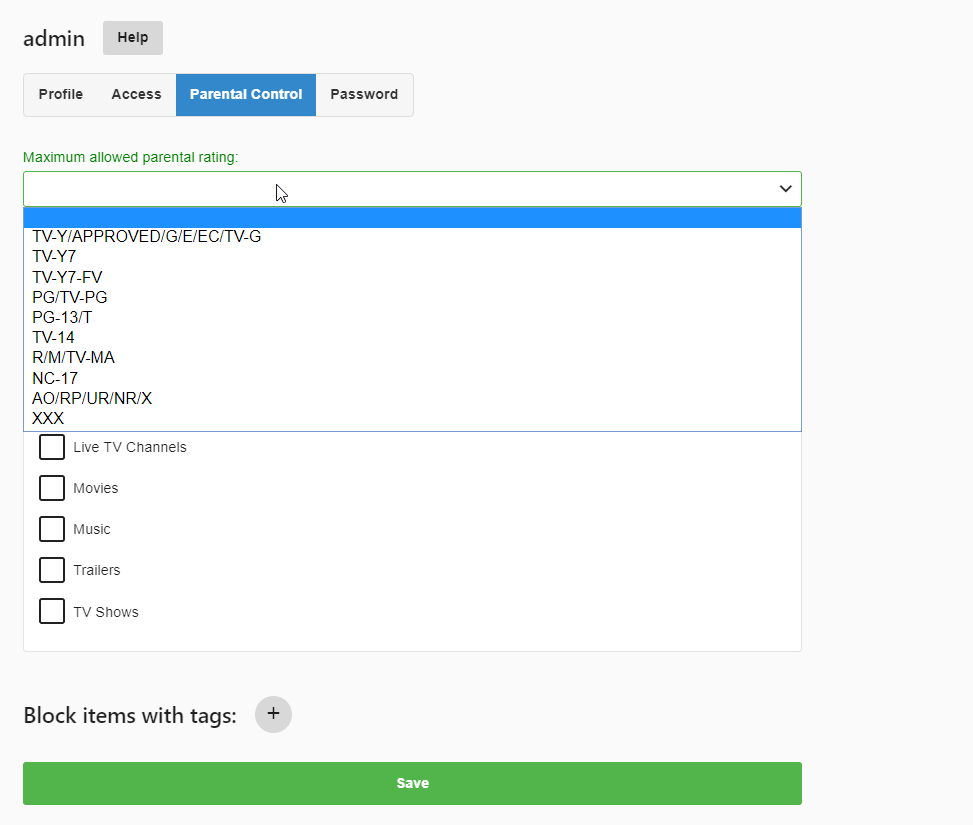The image features a gray background and is part of an interface layout, likely for a profile or account settings page. The top left corner prominently displays the word "Admin." To the right of this, a dark gray sidebar is present, organizing various options. The sidebar includes buttons labeled "Help," "Profile," "Access," "Parental Control," and "Password." 

Beneath these options, the section titled "Maximum Allowed Parental Rating" is shown. This section includes a drop-down menu with various ratings listed inside. The ratings are as follows:

- TV-Y / APPROVE / GE / TV-G
- TV-Y7
- TV-Y7-FV
- PG / TV-PG
- PG-13 / T
- TV-14
- R / M / TV-MA
- NC-17
- AO / RP / UR / NR / X
- XXX

This menu is likely used for setting parental controls, allowing the administrator to specify the highest content rating permitted.